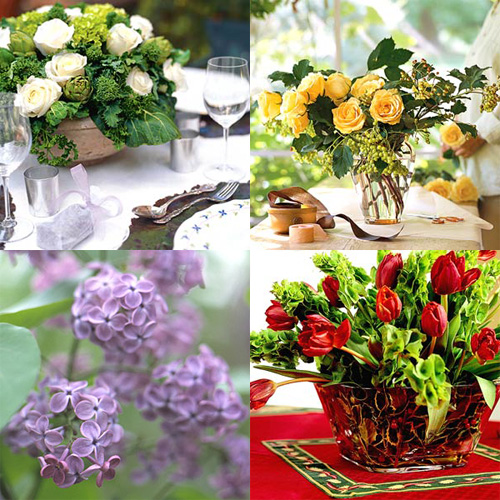This image is a composite of four vibrant flower photos arranged in a larger square, each quadrant showcasing a different floral arrangement. The top left square features a fancy dining table set with china plates, silver cutlery, long-stemmed glasses, and a white tablecloth. The centerpiece is a decorative tan bowl filled with white roses, green leaves, and baby artichokes, or possibly kale. The top right square shows a glass vase filled with water and yellow roses, set on a tabletop covered with white wrapping paper, scattered with ribbon and scissors, hinting at a floral preparation scene. The background has more roses and greenery bathed in sunlight, with hands carefully arranging flowers. In the bottom left square, there's a close-up of light purple flowers, likely lilacs, arranged outdoors under the sunlight, with a sharply focused flower in the foreground and a blurred background enhancing its aesthetic appeal. Finally, the bottom right square depicts a red tablecloth adorned with a rectangular glass bowl full of red tulips and light green leaves, creating a vivid, layered floral composition.